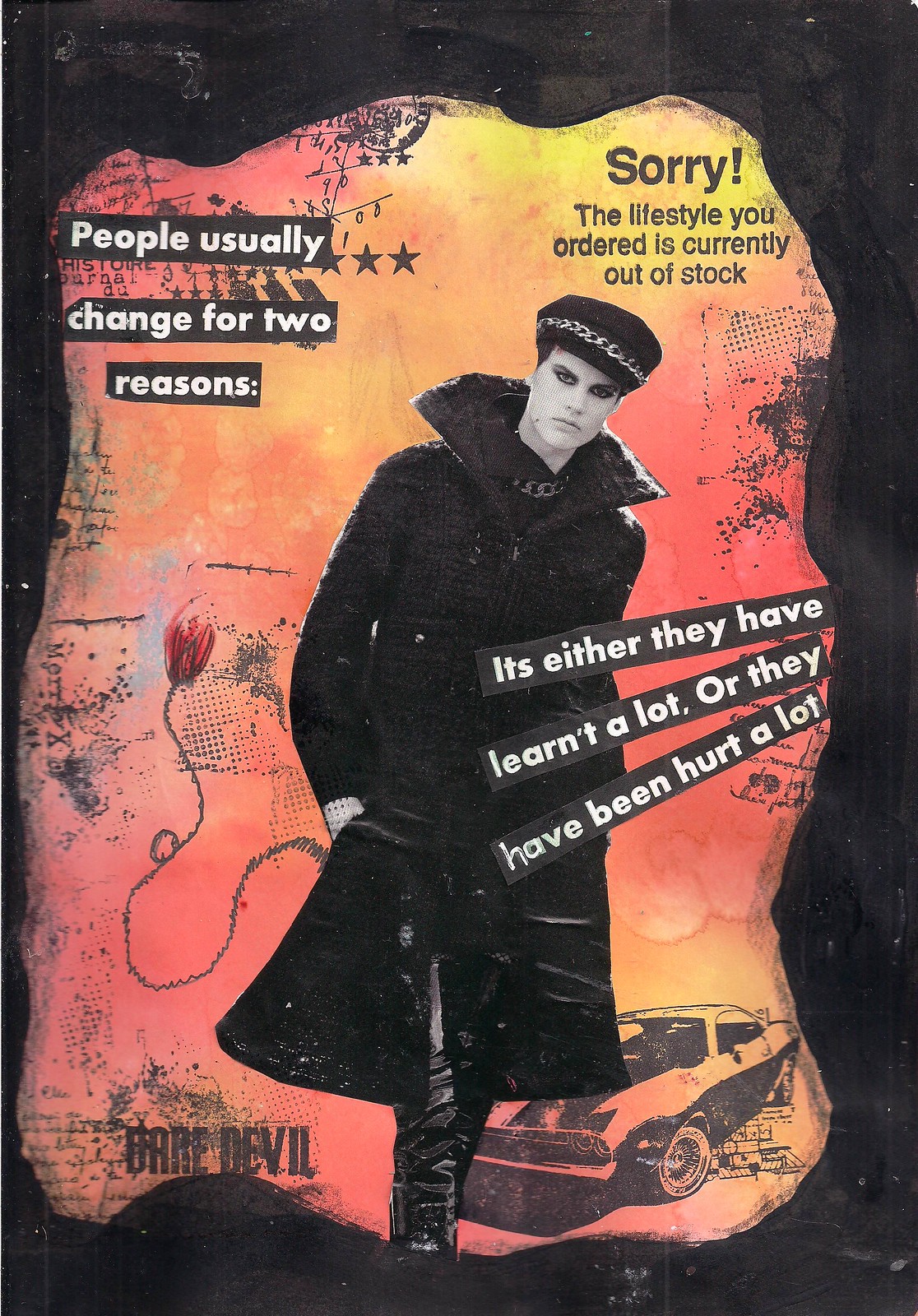The image appears to be a striking, all-black flyer or poster. Dominating the center is a conspicuous red, orange, and yellow splash of color. In the upper right-hand corner of this vibrant burst, bold black letters state, "Sorry, the lifestyle you ordered is currently out of stock." In contrast, the upper left-hand corner features a thought-provoking message in white letters: "People usually change for two reasons." 

Positioned centrally is a tall, white male figure—symbolically depicted in faded black and white—draped in a long black leather trench coat and matching leather pants. He wears a black hat adorned with a chain and thick black eyeliner and dark eyeshadow, enhancing his dramatic appearance. Beneath his coat, a black shirt with a chain around it is faintly discernible. Surrounding him, the backdrop's fiery hues starkly contrast his monochrome presence.

Floating around the figure are three lines of text, each outlined in black bars, with white lettering that reads, "It's either they have learned a lot or they have been hurt a lot."

Adding a nostalgic touch, an illustration of a 1960s Chevy Camaro or a similar sports car can be found at the bottom. In the lower left-hand corner, the word "Daredevil" appears in black letters, adding an air of rebellion and boldness to the overall composition.